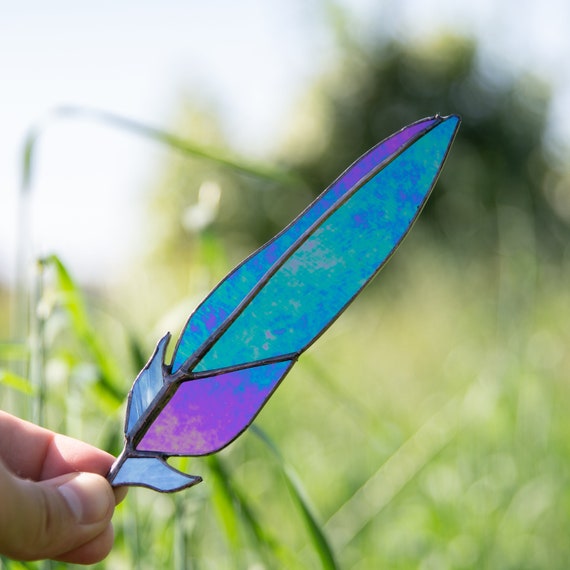The photo captures an up-close, diagonal view of a stained glass feather held by a well-manicured hand from the base. The feather, styled after a goose feather, features a color gradient from turquoise blue at the top to a purplish hue at the bottom and is segmented into five sections. It has a black spine and a black outline that define its structure. The background is blurred, revealing hints of a sunny day with green vegetation, possibly grass, emphasizing the feather's vivid colors and intricate design. The sunlight enhances the metallic sheen of the feather, making its colors pop against the soft focus of the natural scenery behind it.